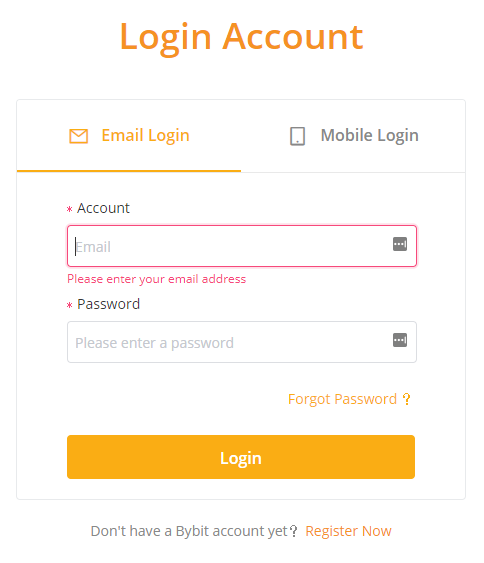This image captures a login screen displayed on a mobile phone. At the top center, "Login Account", printed in bold orange letters, serves as the heading. Below this header, there is a rectangular input area outlined with a faint gray border and filled with white.

The first prompt within this area is for an "Email Login", indicated by an orange line beneath the text and accompanied by an envelope icon, also in orange. Adjacent to this section, "Mobile Login" is written in gray, along with an icon of a cell phone.

Directly below, the word "Account" appears, marked with a red asterisk, signifying a required field. A bordered box outlined in red is provided for the user to input their email address, which is currently blank. Underneath this field, a message in red reads, "Please enter your email address."

Following the email section is a prompt for a password, also flagged with a red asterisk. The field is labeled "Password" with an instruction below that says, "Please enter a password." 

Towards the bottom, there is a "Forgot Password?" link in orange, accompanied by a question mark. Finally, a prominent orange "Login" button is situated at the bottom of the screen.